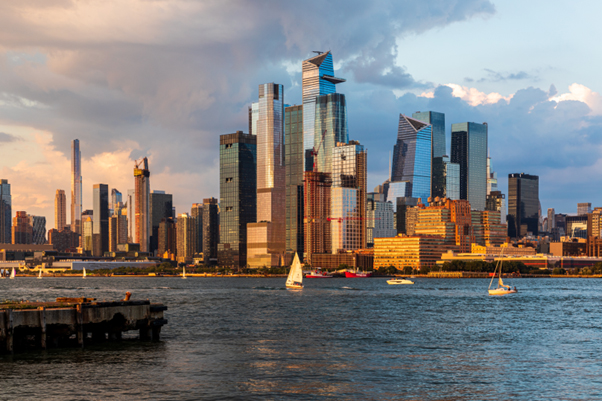This photograph captures an expansive panorama of downtown New York City, likely taken during sunrise or sunset, featuring Hudson Yards and its surrounding skyscrapers. The foreground prominently displays the Hudson River, teeming with sailboats; one sails mid-frame while several more, including one with its sail up, dot the background. A pier extends into the water from the left side. The cityscape is marked by a horizontal line of towering, intricately-shaped glass buildings, with some designs breaking conventional shapes. One exceptionally tall skyscraper in the center boasts a significant ledge. The sky above is a dramatic mix of dark gray and cream clouds, interspersed with patches of blue, adding depth to the vibrant city below.